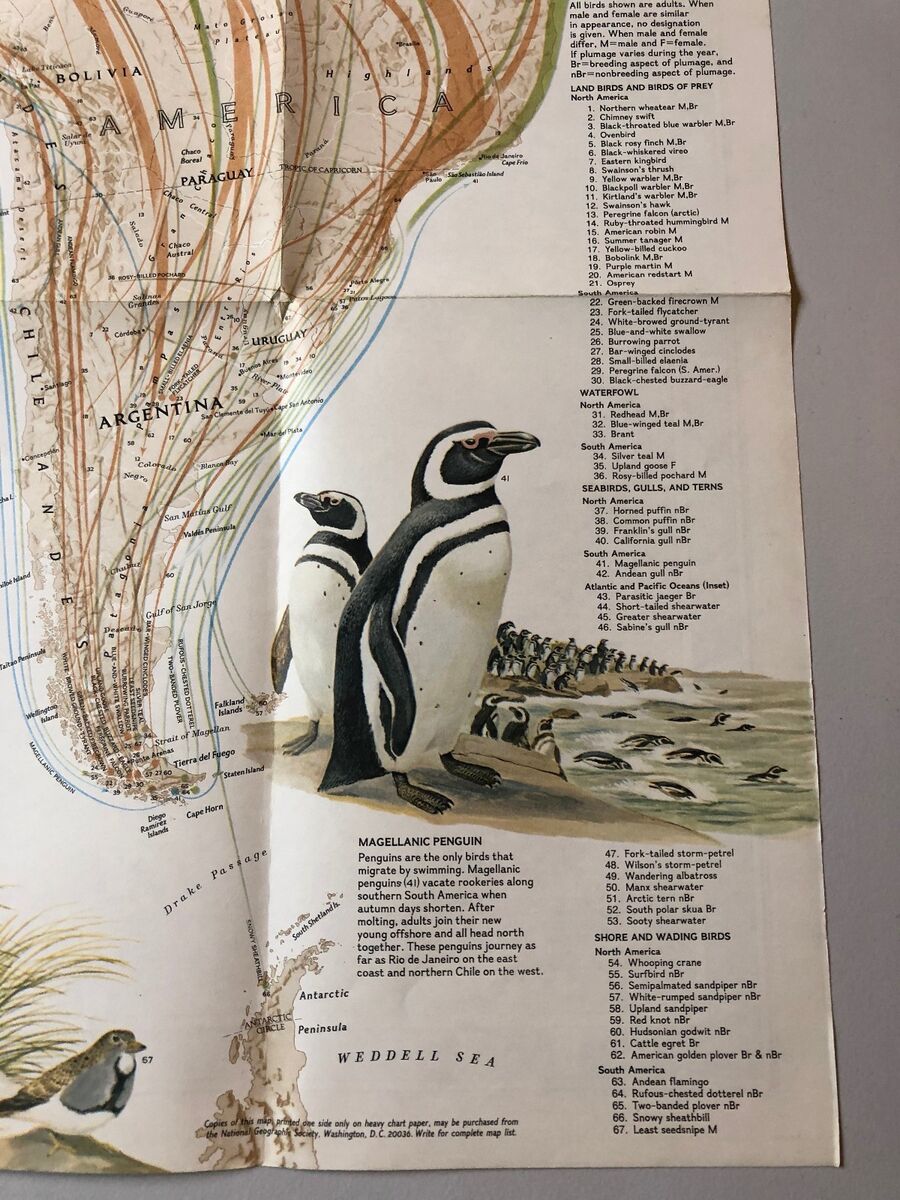The image is a detailed illustrated map of the southern portion of South America, prominently featuring Bolivia, Paraguay, and Argentina. This map is positioned in the top left-hand corner of the image. The central part of the image showcases a pair of large Magellanic penguins, beautifully illustrated and standing out against the backdrop of a bustling colony of penguins diving into the ocean from a beach. Below these primary penguin illustrations, there is descriptive text identifying them as Magellanic penguins. In the bottom left corner, another bird is depicted resting on a rock, while the tip of the Antarctic Peninsula is visible at the very bottom. On the right side of the map, a wealth of information is presented in small black font, likely describing various bird species and their migration routes. Additionally, a section appears to list different categories of birds such as land birds, birds of prey, water birds, seabirds, gulls, and terns, accompanied by small illustrations of these birds. Bird number 41, aligned with the Magellanic penguins, and another bird listed as number 69 are specified, though detailed information on the latter seems incomplete or missing.